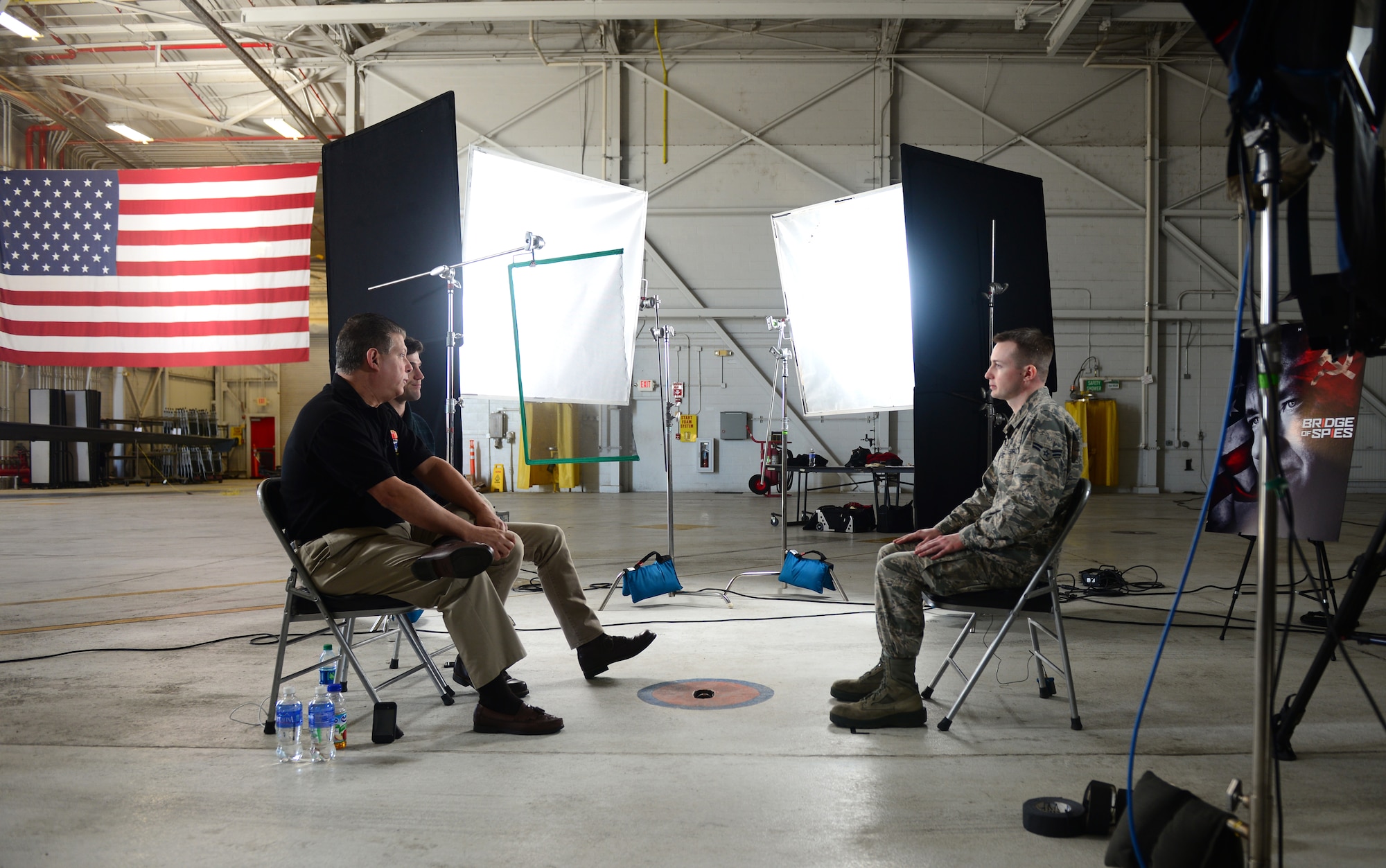The image depicts a color photograph taken indoors, likely in a large building resembling a warehouse or an airplane hangar. The setting is illuminated by numerous bright lights and white reflecting panels, indicating a video or television interview scene. On the right side of the image, a person dressed in camouflage military wear is seated in profile, appearing to be the interviewee. On the left side, two men in civilian attire are seated, interviewing the military individual. Behind them, a large American flag drapes from the ceiling, enhancing the patriotic ambiance. In the background, the expansive space, characterized by its tall ceilings and gray floors, contains various equipment and supplies. Prominently, a camera on a tripod in the right foreground indicates the ongoing recording. Additionally, a "Bridge of Spies" movie poster featuring Tom Hanks is visible on the right, and centrally, four screens arranged in a diamond shape are part of the setup. Water bottles are placed near the interviewers, emphasizing the casual yet professional nature of the scene.